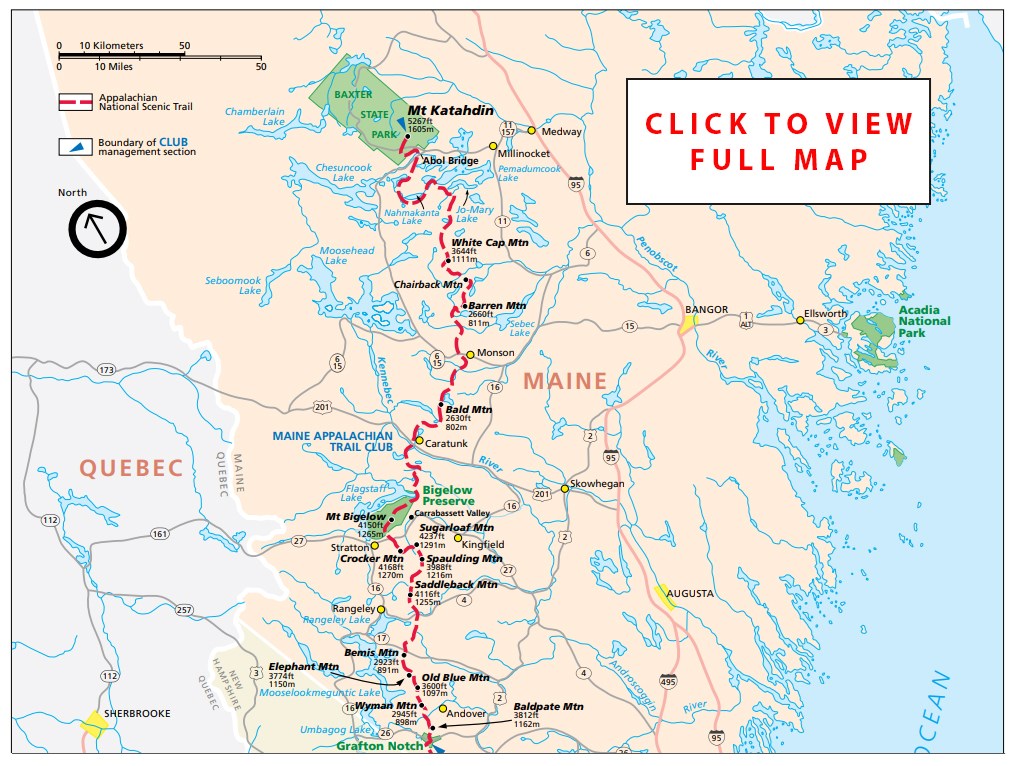This detailed map illustrates the Appalachian National Scenic Trail as it traverses the state of Maine and touches the Quebec border. The red dashed line signifies the Appalachian Trail, winding from Mount Katahdin through Baxter State Park, descending southward through Mount Bigelow and Grafton Notch, and eventually continuing beyond the map's edge. A blue arrow marks the Boundary of Club Management sections. Also prominent are Maine's national parks, including Acadia National Park along the Atlantic coastline, depicted in green. The legend, located at the top left, includes scales in both kilometers and miles for distance reference. The map also highlights various mountains, lakes, and a portion of the ocean, making it a comprehensive tool for hikers and outdoor enthusiasts exploring this region. Additional details emphasize the potential for an interactive experience, encouraging viewers to click to view the full map.